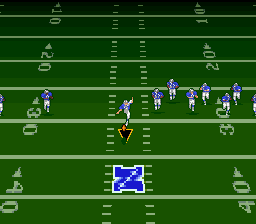This image is a detailed screenshot from an early 90s football video game that likely appeared on classic consoles such as the NES or Super Nintendo. The game features a green football field with horizontal lines marking yard increments from the 10-yard line to the 40-yard line. In this scene, nine players are visible, positioned in a kickoff formation around the 30-yard line. The players are wearing blue jerseys with white pants and gray helmets. At the center of the screen, a kicker is actively engaged in kicking the football. Toward the bottom of the screen, the field prominently features a large, blue capital "N" with a diagonal line running from the top right to the bottom left of the letter. The game does not explicitly identify the team, though the uniforms might evoke imagery of the Detroit Lions. The field and its markings fade to black as they approach the top of the screen, setting the visual context for an early-generation football video game.